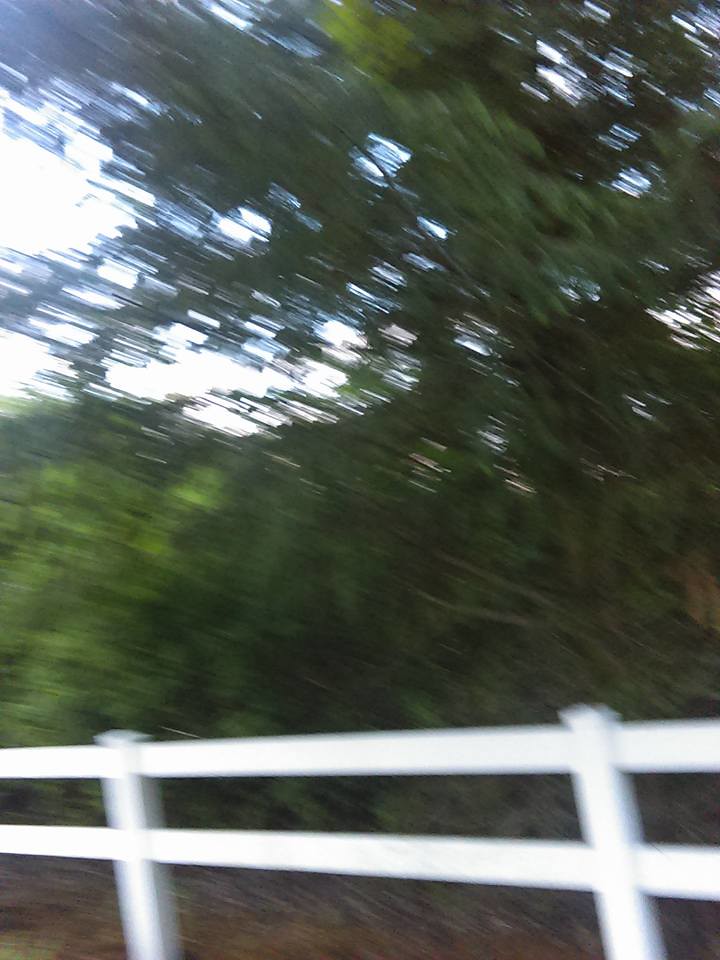In this very blurry photograph, the setting appears to be alongside a road bordered by a white wooden fence with two horizontal bars and vertical posts. The foreground features this distinct fence style. Beyond the fence, there are green, leafy trees that fill most of the background. The photo was evidently taken while the camera was in motion, resulting in streaky imagery, particularly noticeable in the upper left corner. Through the trees, patches of blue sky and white clouds are visible. The bottom of the picture shows a hint of pine needles scattered on the ground, adding to the natural ambiance of the scene.